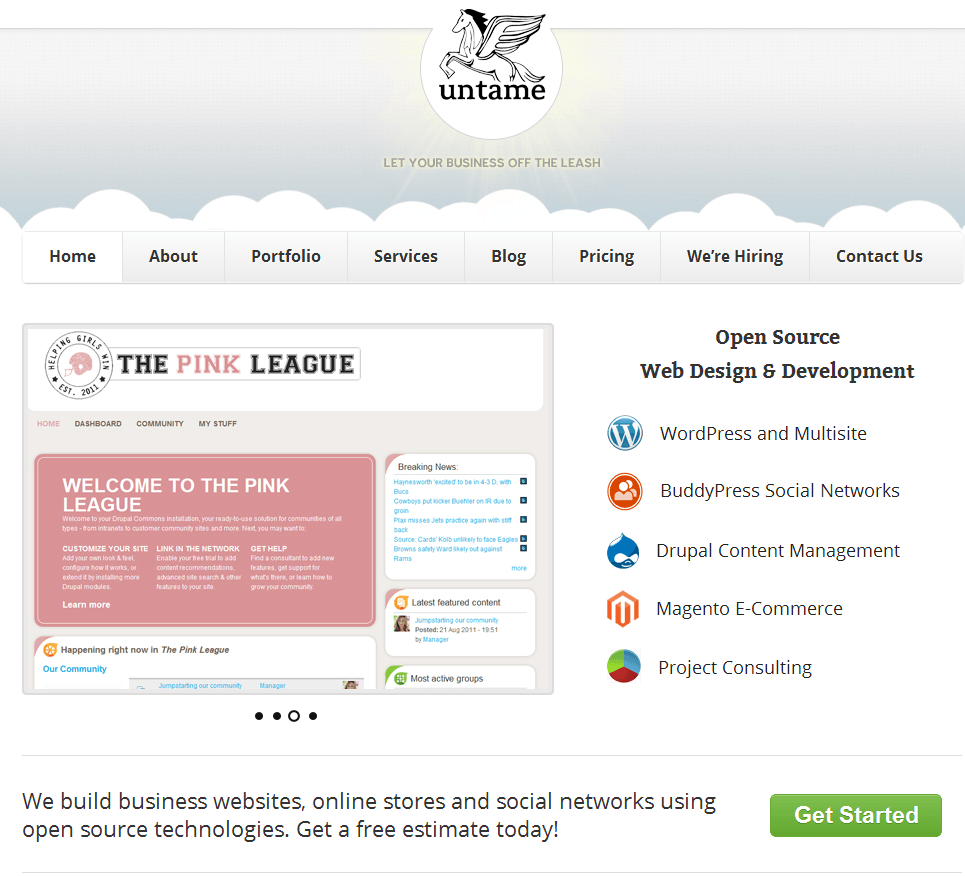In the center top section of the image is an illustration of a Pegasus with the word "Untame" below it, styled in a typewriter font. The background features a gradient of hazy blue, pink, and yellow hues, transitioning from the top to the middle. The Pegasus is rendered in a black outline, creating a striking contrast against its backdrop. Encircling the Pegasus is a white cut-out, forming an incomplete circle with the top segment missing.

Beneath the word "Untame," there is a tagline in gray font that reads, "Let your business off the leash." Below this, fluffy white clouds span the entire width of the image, forming a visual divider.

Further down, there is a navigation bar with buttons labeled "Home," "About," "Portfolio," "Services," "Blog," "Pricing," "We're Hiring," and "Contact Us." The "Home" button is highlighted in white, indicating that this is the currently active page, while the other buttons are shown in an off-white color.

On the bottom left, there is a section for "The Pink League," featuring a logo of a pink football helmet inside a circle. Below the logo, text states, "Helping girls win, established 2011." Beneath this, a navigation menu includes options such as "Home Dashboard," "Communities," and "My Stuff." There is a welcome message to the Pink League digital community, mentioning it is built on the Drupal Commons platform, which is a ready-to-use solution for various types of communities. Further options are provided to customize the site, link within the network, and seek help.

On the right side of the image, additional content is likely present, but it is not fully visible in the provided description.